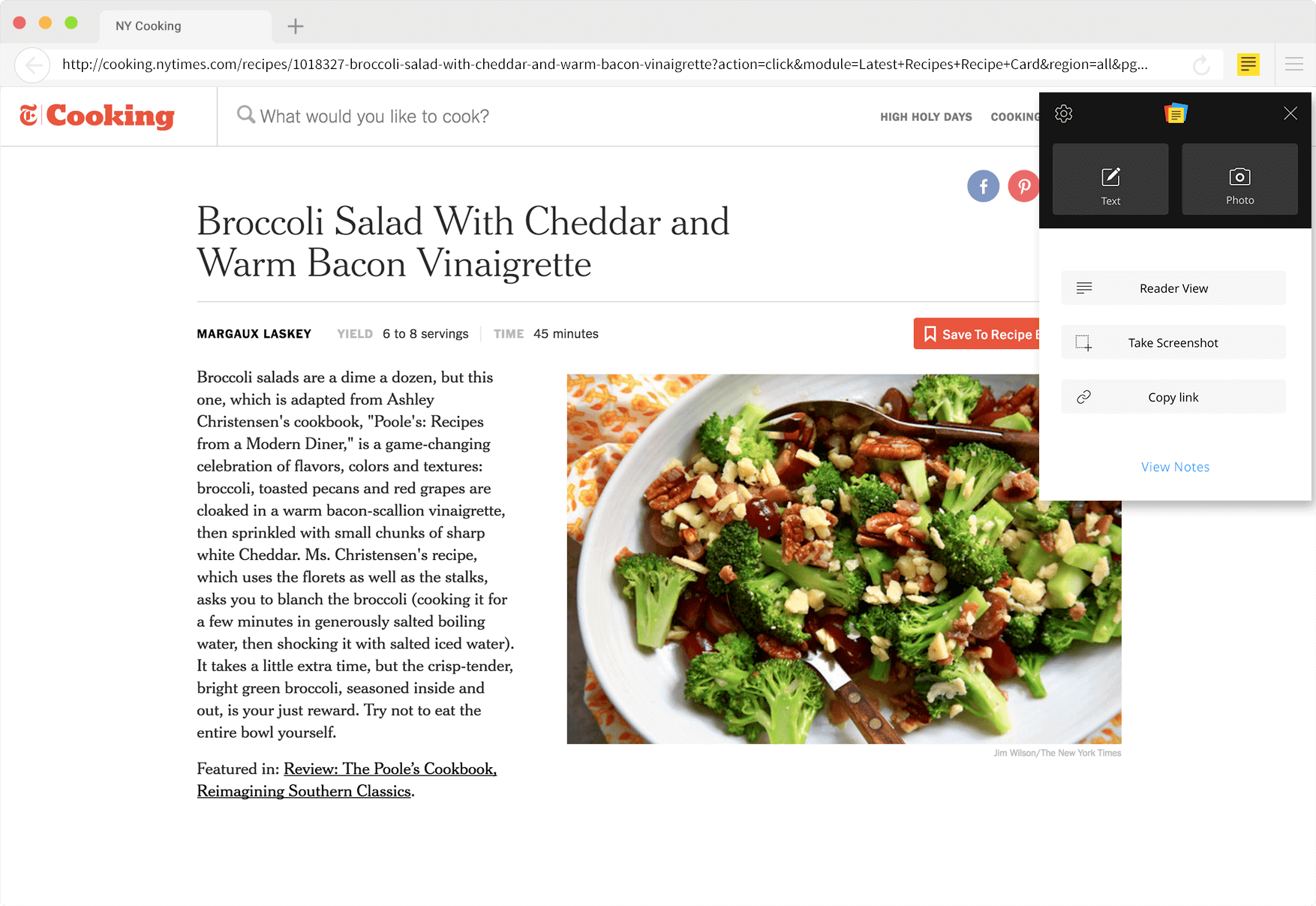This is an image of a webpage with distinguishing features. At the top left, there are three colored circles: a red circle, a yellow circle to its right, and a green circle further to the right. Due to the low quality of the image, the webpage link itself is blurry and the text is difficult to read. The overall resolution of the image is noticeably poor, making details hard to discern. 

In the top left corner, "cooking" is written in a red font. To the right of this text, there is a search bar with the placeholder text "What would you like to cook?" Immediately below, there is a recipe title that reads "Broccoli Salad with Cheddar and Warm Bacon Vinaigrette." 

Toward the bottom and on the right side of the image, there is a picture of a plate of food, encircled by a white rim, showcasing various vegetables.